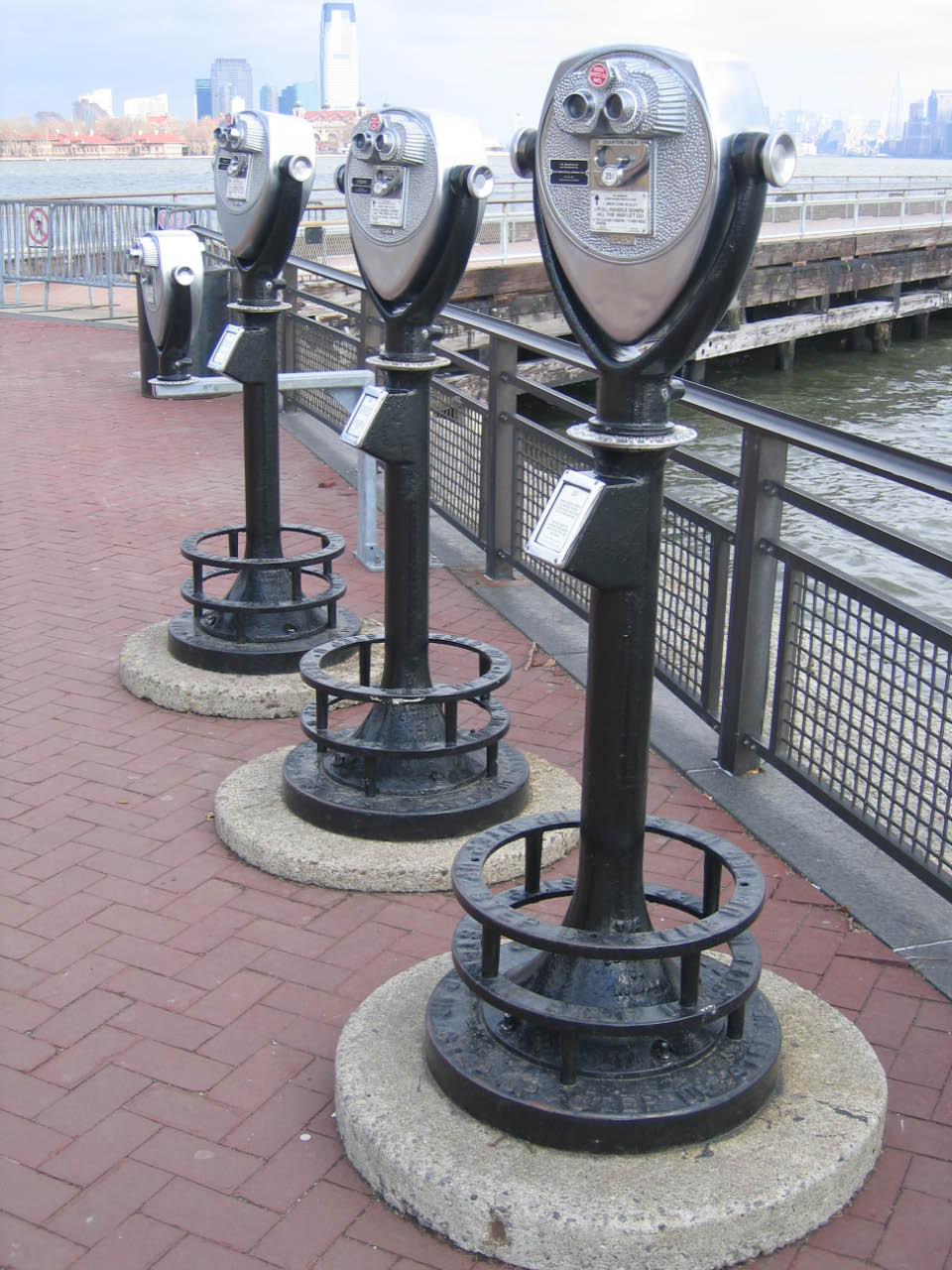This photograph captures an overcast day by the edge of a broad body of water, possibly a bay, river, or lake, with the smoggy skyline of an unidentified city in the distant background. Dominating the foreground are three coin-operated binoculars, designed for sightseeing, their steel-colored tops mounted on black poles with black foundations anchored to round concrete bases. A red brick walkway leads up to these binoculars, bordered by a grid-like black guardrail that angles from the upper left to the bottom right of the image. The scene suggests a popular tourist spot, enhanced by the presence of additional guardrails for safety.